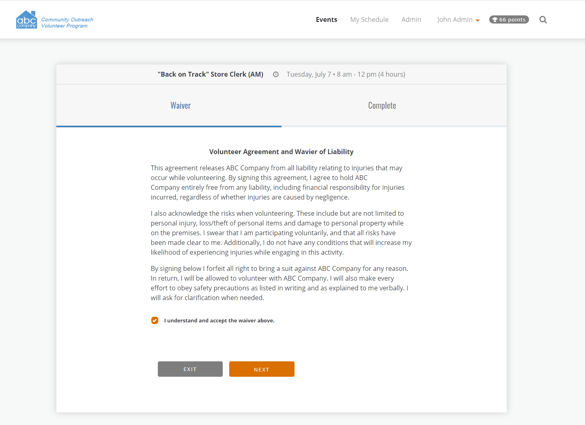**Screenshot of the 'Community Outreach Volunteer Program' Event Page on ABC Company's Website**

The image showcases a screenshot of a web page dedicated to the Community Outreach Volunteer Program on the ABC Company website. At the top of the page is a white header featuring a blue house logo with the letters "ABC" in white text. To the right, the header displays the title "Community Outreach Volunteer Program" in blue text.

On the right side of the header, there are several navigation options, with "Events" highlighted in bold text, indicating it is the selected section. Adjacent to this, lighter gray text displays additional menu options: "My Schedule," "Admin," and "John Admin." An orange downward arrow is positioned to the right of the last menu option.

Beneath the header, a pop-up window is visible. This window has a light gray header titled "Back on Track, Store Clerk (AM)" aligned to the left, accompanied by a medium gray circle. To the right, light gray text provides the event details: "Tuesday, July 7, 8 AM to 12 PM (4 hours)."

Within the pop-up body, there are two selectable tabs. The first tab, labeled "Waiver," is highlighted in blue and underlined, while the second tab, "Complete," is shown in thick gray text. Below these tabs, the main content of the pop-up is presented against a white background.

At the top of this section, bold text announces the "Volunteer Agreement and Waiver of Liability," followed by three paragraphs in thin gray text. These paragraphs contain the legal language of the waiver, releasing ABC Company from liability for injuries incurred while volunteering, acknowledging the risks involved, and affirming that the volunteer is participating voluntarily and understands all safety precautions. The agreement also states that by signing the document, the volunteer forfeits the right to sue ABC Company in exchange for the opportunity to volunteer.